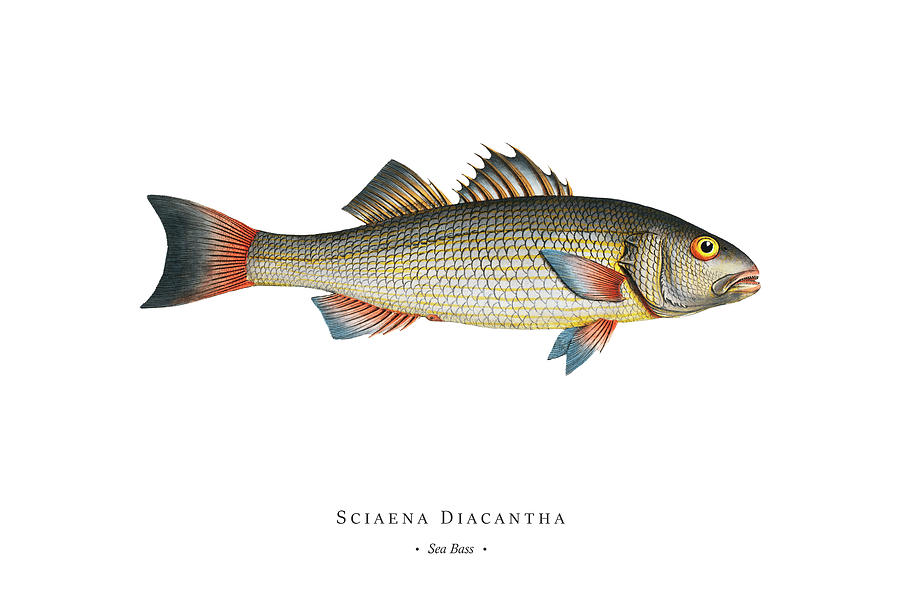This image is a detailed, brightly colored scientific illustration of a sea bass, labeled "Cyana diacantha" in small print at the bottom, with "sea bass" in even smaller print below that. The fish is set against a plain white background, emphasizing its vivid details. It is facing to the right, showcasing a long, plump body adorned with yellow and silver scales that fade to a grayish-brown towards the top and yellow-beige on the underbelly. The fish features a distinctive, slightly open mouth with a pink hue and a striking large yellow eye rimmed with orange.

The fins are a highlight of the artwork, with the tail fin being red tipped with blue, and the bottom fin sharing this red and blue pattern. The top dorsal fin stands out with its yellow and silver coloring, complemented by a pointy fin next to it with a gold and silver hue. Smaller fins near the head also display a red and blue pattern. In total, the fish exhibits seven intricately colored fins. The detailed scales and vibrant coloration make this scientific illustration reminiscent of the classic Audubon style, bringing the sea bass to life in stunning detail.